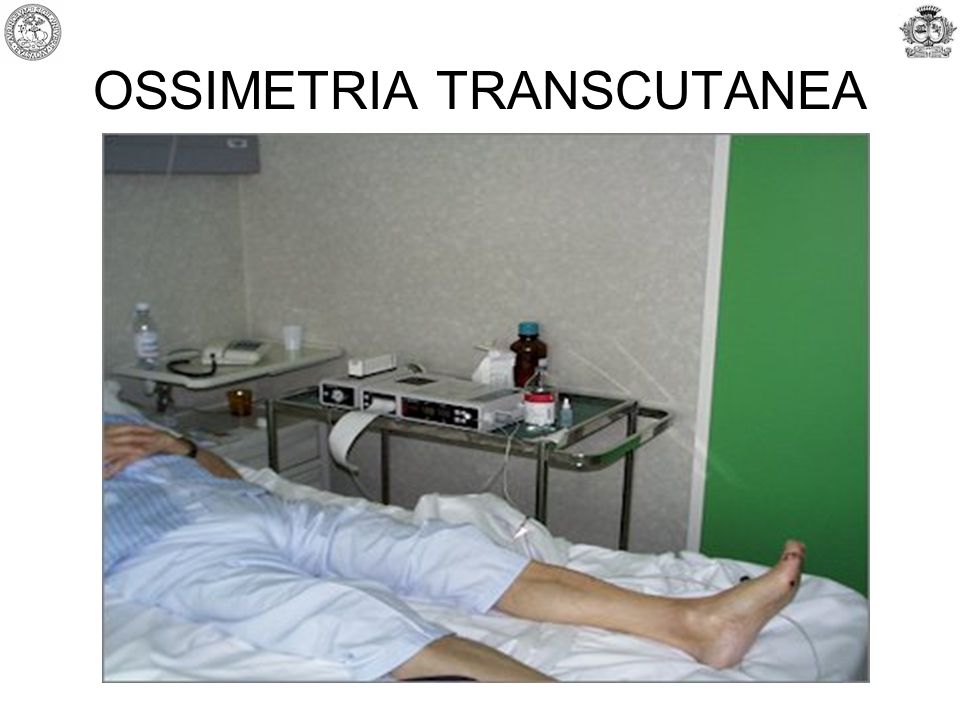The photograph depicts a hospital setting with a patient lying in a bed, visible from mid-torso downward. The individual is wearing a shirt with blue and white stripes, and their toes are pointing upwards, indicating they are supine. Their hands, featuring a black watch, are crossed over their chest. The bed is covered with a white sheet that is pulled up to their mid-thigh. Adjacent to the bed is a metal table holding a gray box with wires extending from it, suggesting medical equipment, possibly an EKG machine. Next to the box are a clear bottle with a white label and an amber-colored bottle that might contain juice, potentially cranberry. On the same table, a dated telephone, another plastic bottle, and a white cup are visible. The walls in the background feature a white-speckled gray color, transitioning to a bright green on the right side. Above the green section, black text reads "OSSIMETRIA TRANSCUTANEA," along with a small, indistinct emblem in the upper right corner, giving the impression that this is an older, non-American hospital room.